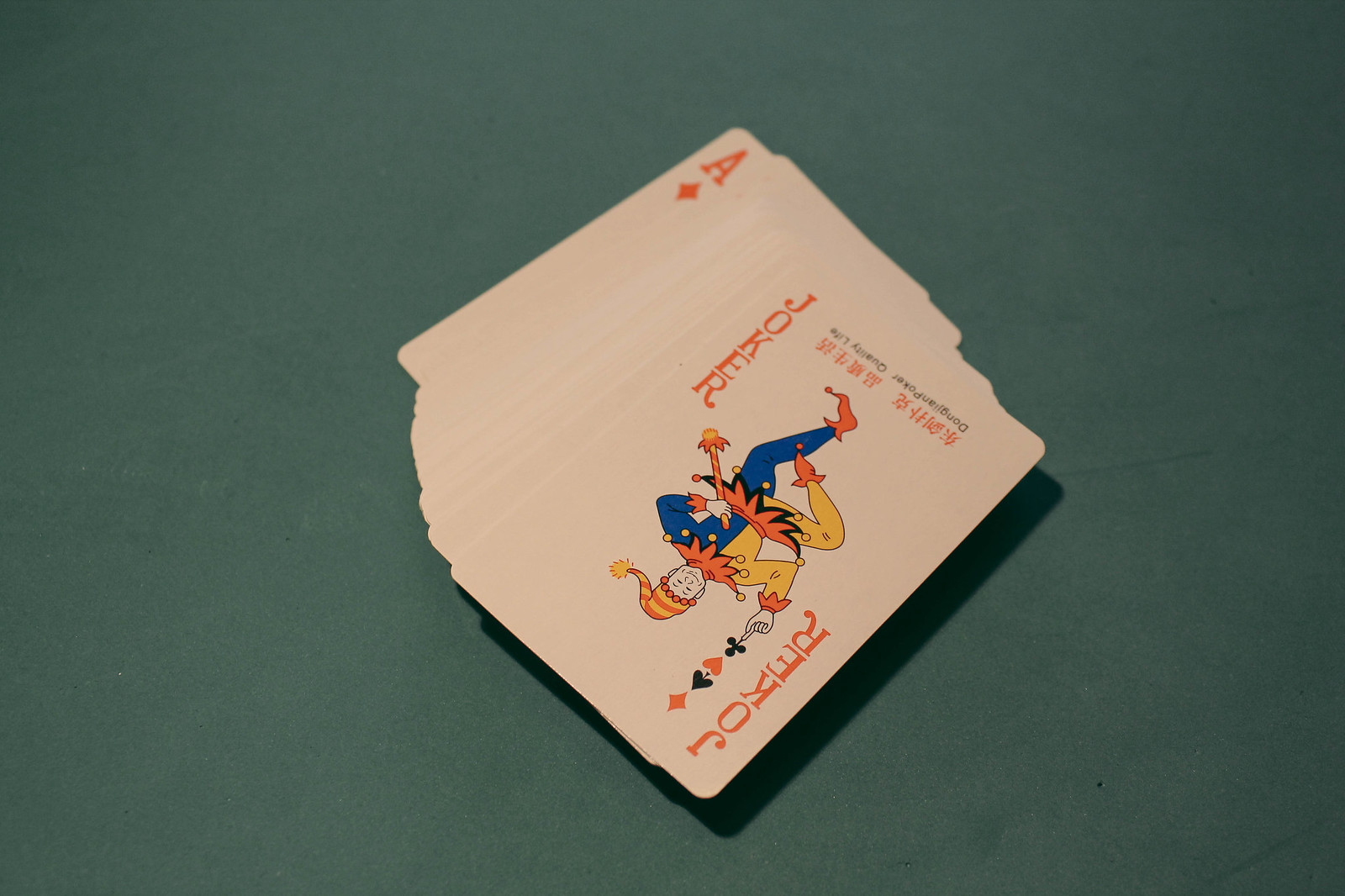In this image, a stack of playing cards is arranged in a semi-fanned out formation, creating a three-dimensional effect as they rise off the table. Despite the fan, the faces of the cards remain largely obscured, except for the top card, which is a Joker, and the bottom corner card, which is the Ace of Diamonds. The background features a rich hunter green, velvet-like fabric reminiscent of a pool table, marked with subtle lines likely from the cards being moved across its surface. The Joker card displays a vibrant court jester, with a costume split into blue and yellow halves, accented by orange and yellow neck and waist details, and orange shoes. The jester holds one finger aloft, balancing the symbols of clubs, hearts, spades, and diamonds in a whimsical, stacked arrangement. The playing cards themselves possess a slightly off-white hue, adding to the timeless appeal of the scene.